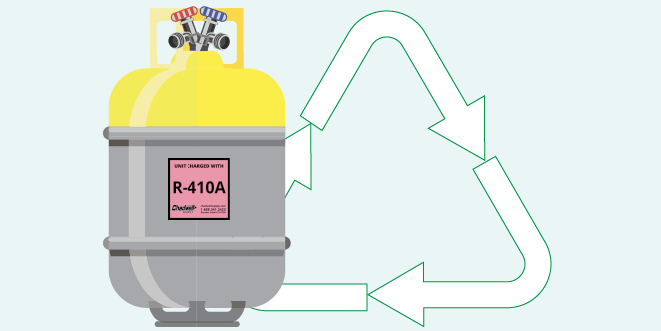The image features a wide, dull light green background that evokes an environment-friendly feel. On the left side of the image is a square-shaped tank with a yellow top third and a gray bottom two-thirds. The tank has a distinct yellow handle and two nozzles at the top, colored red and blue, with projections that suggest connections for pipes or hoses. The nozzles have circular screw caps typically used to open and close the valves. Additionally, a lighter gray stripe curves around the tank's sides. Attached to the tank's front is a prominently placed pink sticker that reads "R-410A" in large black letters, though further text is too small to discern. The tank stands on a base resembling two U-shaped supports with a flat portion underneath. To the right of the tank and slightly behind it, a recycling symbol made up of three white arrows bending around to form a triangle with a medium green outline is visible, further emphasizing the eco-friendly theme of the image.